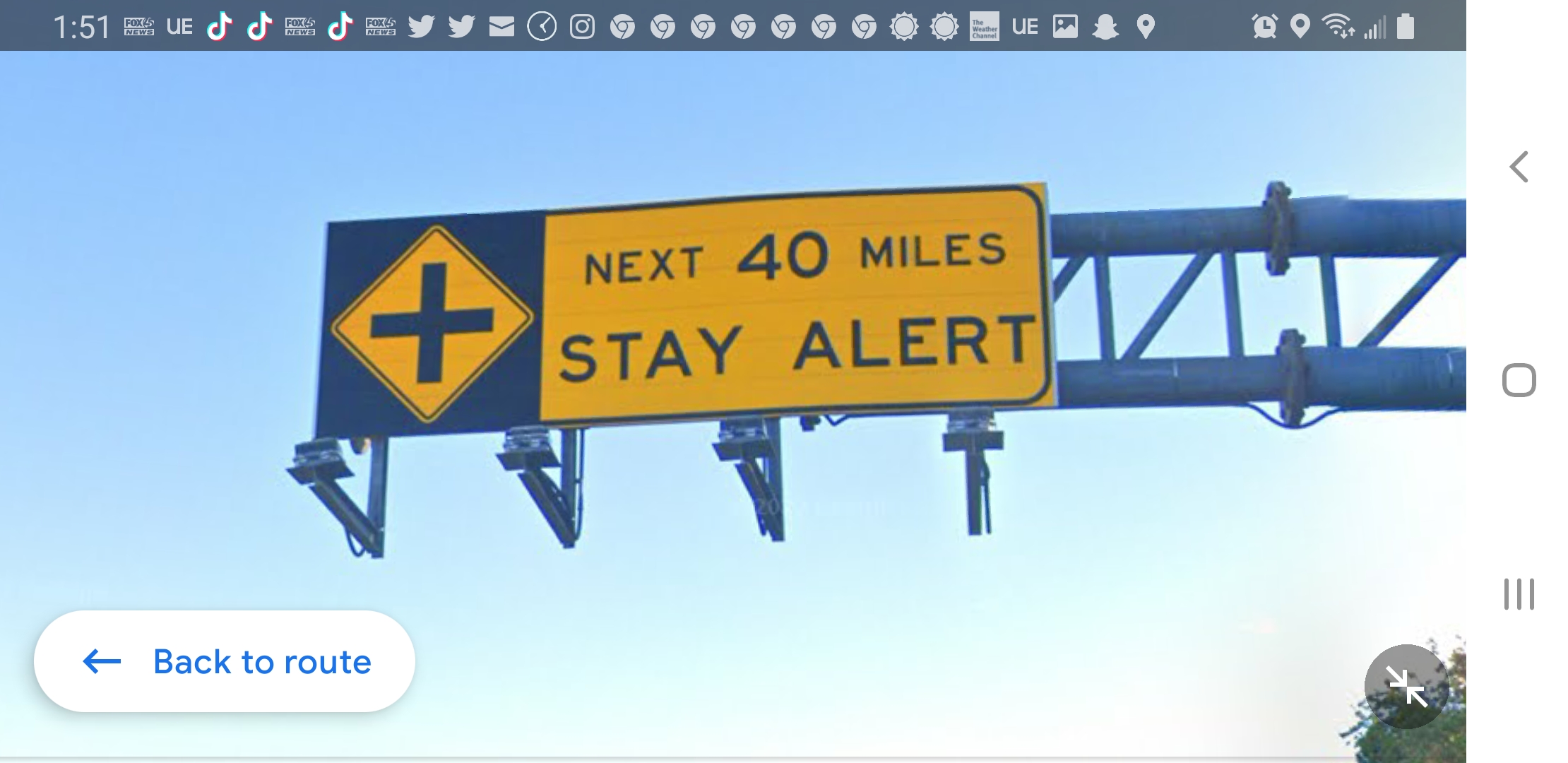This image, likely taken on a smartphone, captures a detailed scene emphasizing road safety. At the top of the photo, there is a typical smartphone interface display showing various icons such as the clock, notifications from TikTok, Twitter, Chrome, and Snapchat, along with indicators for cell signal strength, an alarm, and battery percentage. The main focus of the photo is a road sign mounted on a high pole, extending horizontally over the roadway. The sign, in striking yellow and black colors, features a cross symbol representing an intersection and carries a cautionary message: "Next 40 miles, stay alert." The pole also supports four lights that would presumably illuminate the sign at night. The photo is taken during daylight, emphasized by the clear blue sky serving as the backdrop.